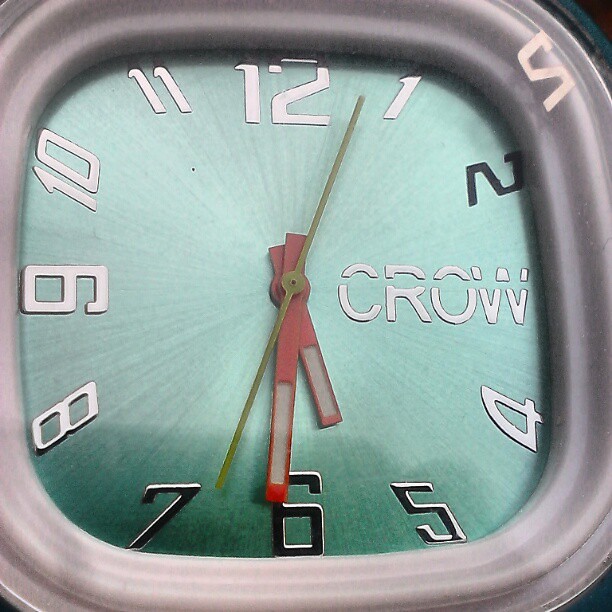This photograph captures a close-up view of a square-shaped clock with a distinctive design. The face of the clock is a soothing light teal color, contrasting with its numerals which are mostly white. Interestingly, the numbers 2, 5, 6, and 7 stand out in black. The clock features a golden dial, complemented by two red hands indicating the time, which is set at 5:30. The clock’s outer frame is a slightly circular square, finished in a sleek silver color, adding a modern touch to its overall appearance.